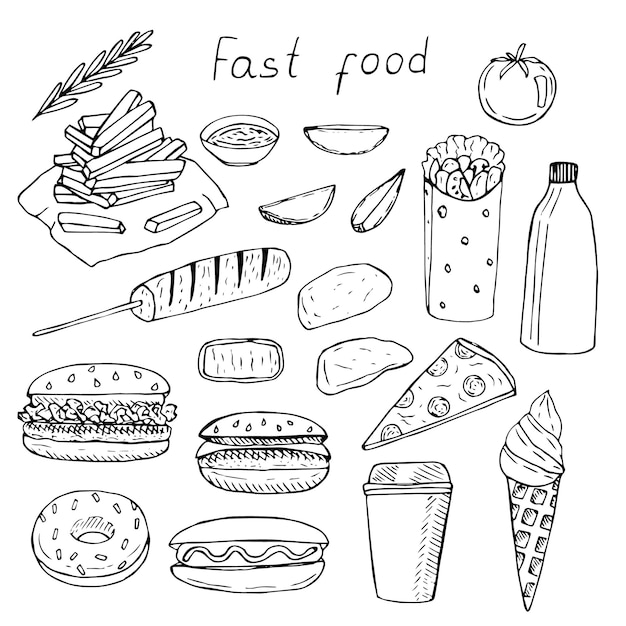The image showcases a detailed black and white drawing, either hand-drawn or computer-generated, featuring a variety of fast food items on a completely white background. Titled "fast food" in a basic handwritten style at the top, the drawing includes an array of iconic American foods. You can see a hamburger or chicken sandwich, a hot dog, a corn dog, a slice of pizza, potato wedges, and a container of french fries with a dipping sauce. There are also sweets like a donut and an ice cream cone, and beverages like a glass of milk and a mug of coffee. Additionally, the illustration depicts a tomato, a rosemary leaf, possibly a lettuce wrap, and what looks like barley in the upper left corner. The entire composition is rendered with minimal shading, giving it a simple yet comprehensive portrayal of classic fast food items.